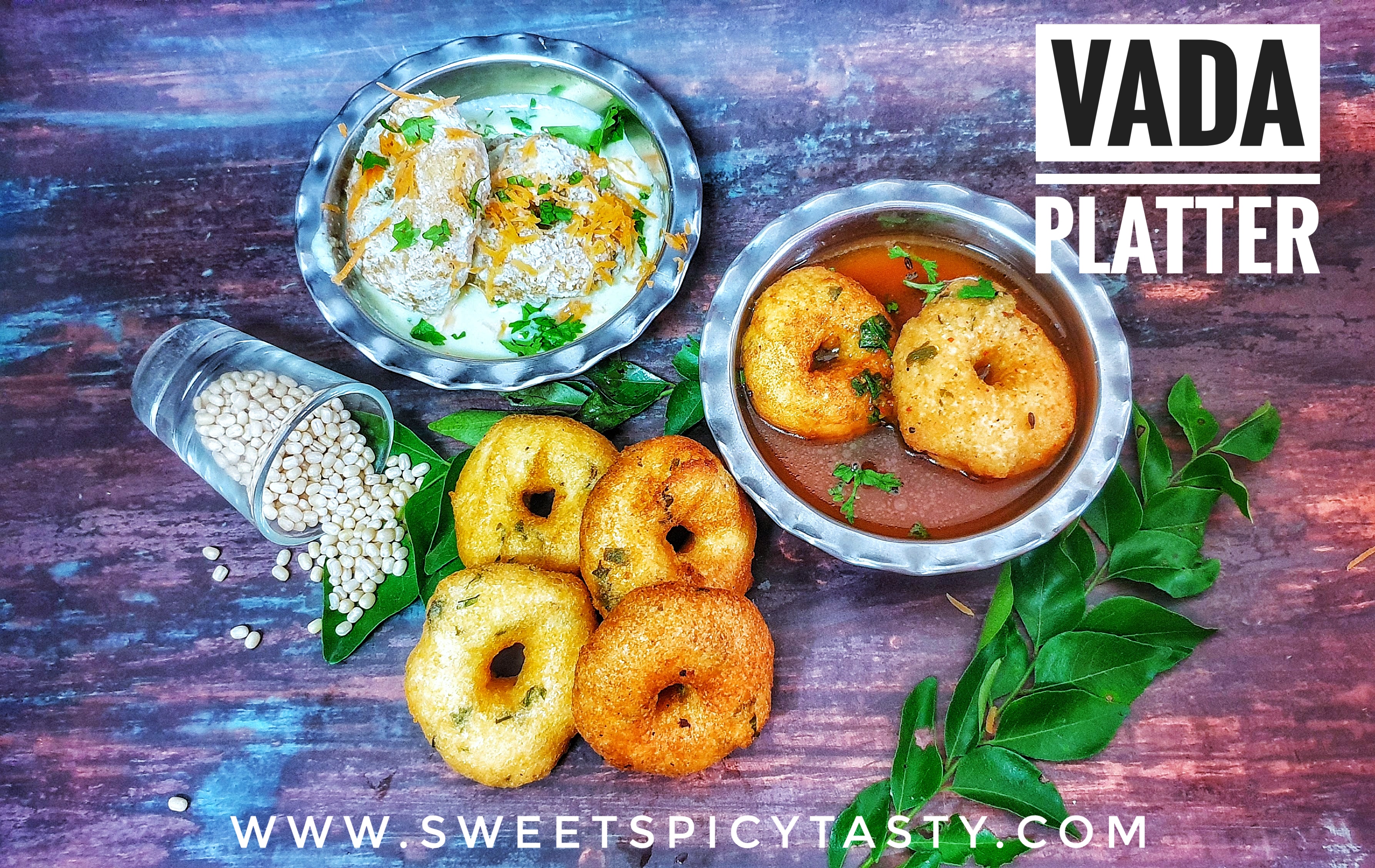The image is a detailed advertisement for a website, www.sweetspicytasty.com, featuring a "VADA PLATTER." Set on a rustic wooden table with shades of blue and purple, the composition includes various elements meticulously arranged to capture attention. 

At the top of the image, "VADA" is prominently displayed in black letters, followed by a line and "PLATTER" beneath it in bold white text. Centered in the image are two silver platters containing appetizing food items. 

The first platter presents a white food object, potentially potatoes, adorned with yellow cheese-like shavings and garnished with green herbs such as basil or cilantro, all immersed in a creamy sauce. The second platter holds donut-shaped, bagel-looking items, dipped in a rich red sauce, also sprinkled with herbs. 

Adjacent to these platters, a glass cup tips over, spilling beans or seeds onto the table, intermingling with an arrangement of lush green leaves. This vibrant culinary scene is surrounded by a few more of the bagel-donut items, accentuating the overall theme and delicious appeal of the Vada Platter.